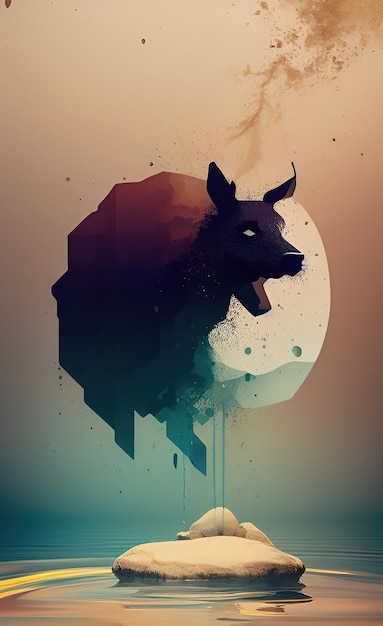The painting is a digitally styled rectangular artwork that vividly captures a fantastical scene. Dominating the composition is a deer-like or moose-like creature, possessing white diamond-shaped eyes and an open mouth as if roaring, its features lending it a demonic aura. Its body and head fill a substantial part of the painting, imposing against a tan background. To the right of this creature is an artistic representation of a moon, colored in a mix of white and blue, with stylized droplets falling from it. These drops cascade onto a prominent rock below, which is flanked by a metallic silver-colored liquid that emits ripples outward. The celestial backdrop also includes abstract gray circles against the moon, enhancing the otherworldly ambiance. The scene is tied together with a palette transitioning from tan to shades of burgundy and blue, creating a surreal and dynamic visual narrative.